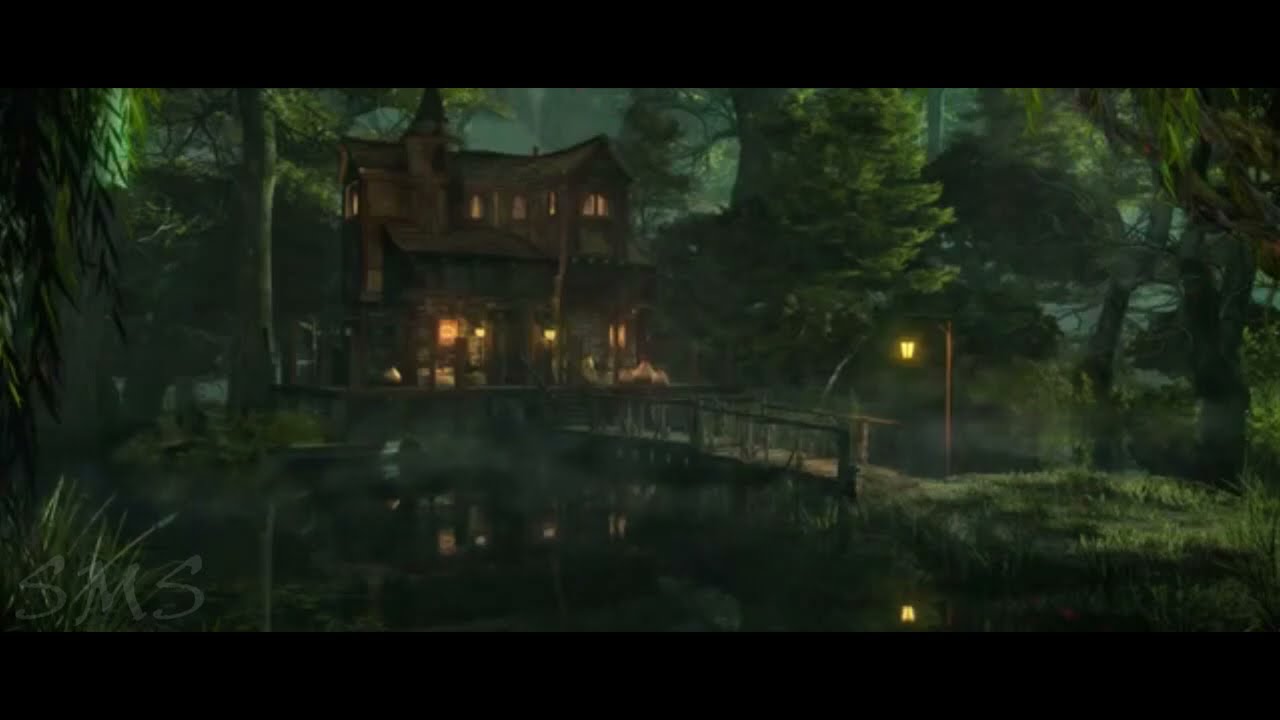This is a wide rectangular image, likely a screen capture of a video game or a digital 3D artwork, featuring a dark and somber nighttime scene. The top and bottom of the image are cropped by black rectangular strips, suggesting it is a screenshot. The scene is set in a dense, deep green forest with thick-leaved trees framing the left and right sides. In the bottom half of the image, a green-tinted body of water reflects the surroundings. A small brown wooden bridge stretches across this water, leading to a large, two-story brown house with lights shining from its windows. The house, located towards the top left of the image, features a prominent turret above its tallest window and is fronted by two glowing lanterns. At the beginning of the bridge, a lamppost with a yellow light illuminates the way. The initials "SMS" are subtly embedded in the forest in the same dark green tone. The overall tone of the image is ominous and uncertain, accentuated by the intricate details of the reflective water, illuminated house, and surrounding dark forest.